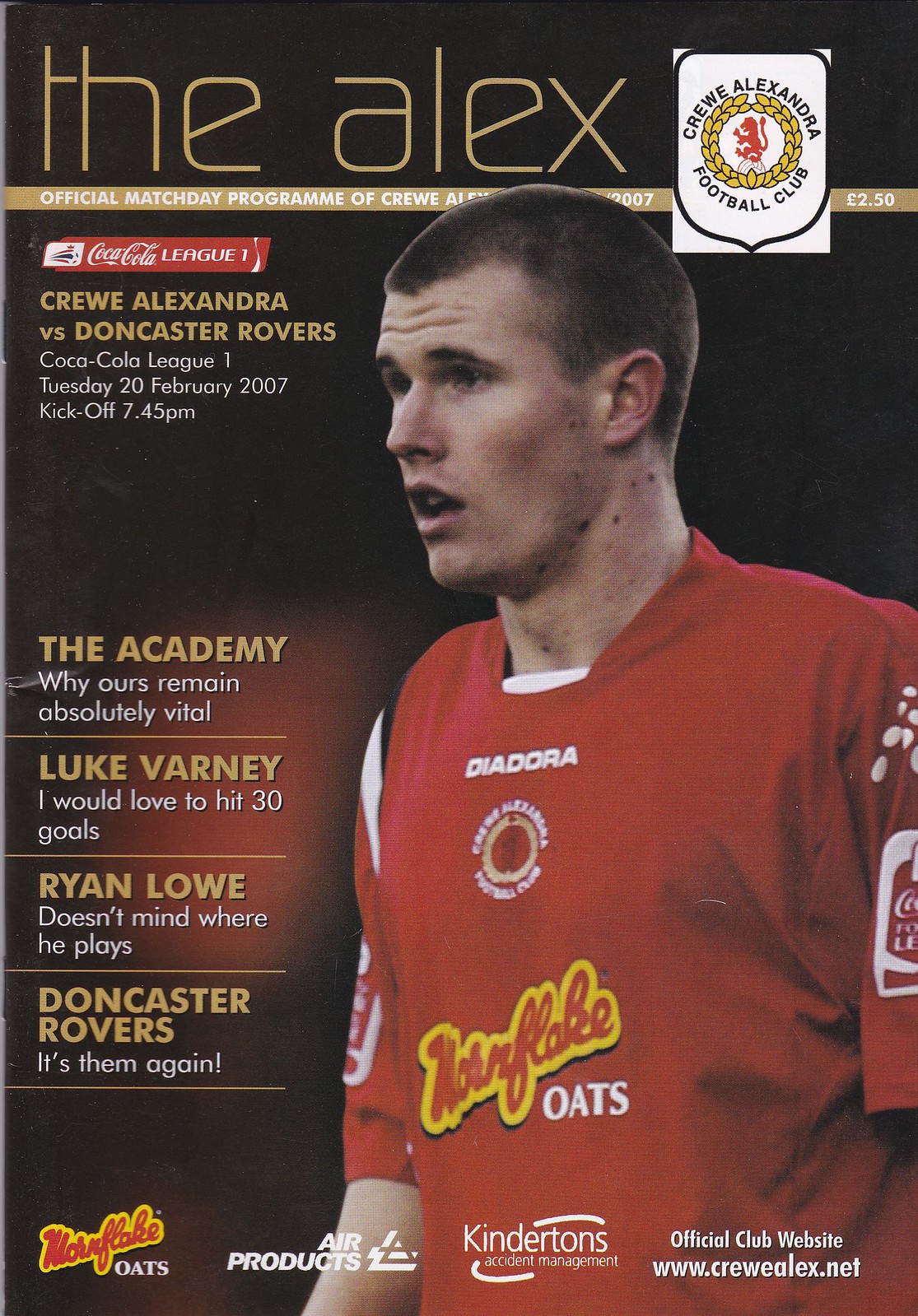The magazine cover features the official match program for Crewe Alexandra Football Club. At the top, "the Alex" is written in lowercase gold font. Below it, a red horizontal box displays the Coca-Cola logo, followed by "League" in white font. Underneath, "Crewe Alexandra versus Doncaster Rovers" is written in gold font, with "Coca-Cola League 1 Tuesday 20 February 2007 kickoff 7:45 p.m." in white font below. On the right side of the image, a man in a red soccer jersey, adorned with multiple sponsor logos, looks surprised towards the left. The bottom of the cover features additional sponsor logos, including Northern North Flake, Morn Flake, Oats, Air Products, and Kinder Tins. The magazine highlights the match and offers features such as information on the Academy.